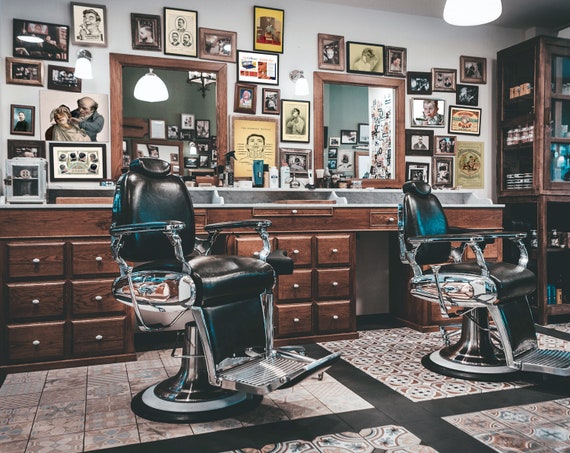The photograph showcases a vintage barbershop, meticulously preserved or recreated to embody the mid-20th-century charm. Dominating the scene are two classic, black leather barber chairs from the 1960s, each featuring silver handles, outward fanning footrests, and circular bases with foot pedals for height adjustment. The floor beneath forms an intricate mosaic with four different tile patterns, separated by black tiled crosses. To the left center of the first chair, tiles are circular and flourished with unique colors and floral designs, while under the right chair, the tiling features brown-cornered circles with small squares, surrounded by a mix of crosses, half circles, and squares.

Behind the chairs, a wooden counter equipped with numerous pull-out drawers and shelves holds various hair-cutting and shaving accessories, including jars for sterilizing combs and scissors. Above the counter, large wood-framed mirrors anchor a wall densely adorned with black-and-white photographs and portraits. These pictures, likely dating back to the 1950s or 60s, depict a plethora of hairstyles and client snapshots. On the far right, a cabinet stores additional barber supplies and possibly products for sale. The image evokes a nostalgic atmosphere, capturing the essence of a bygone era in barbering.